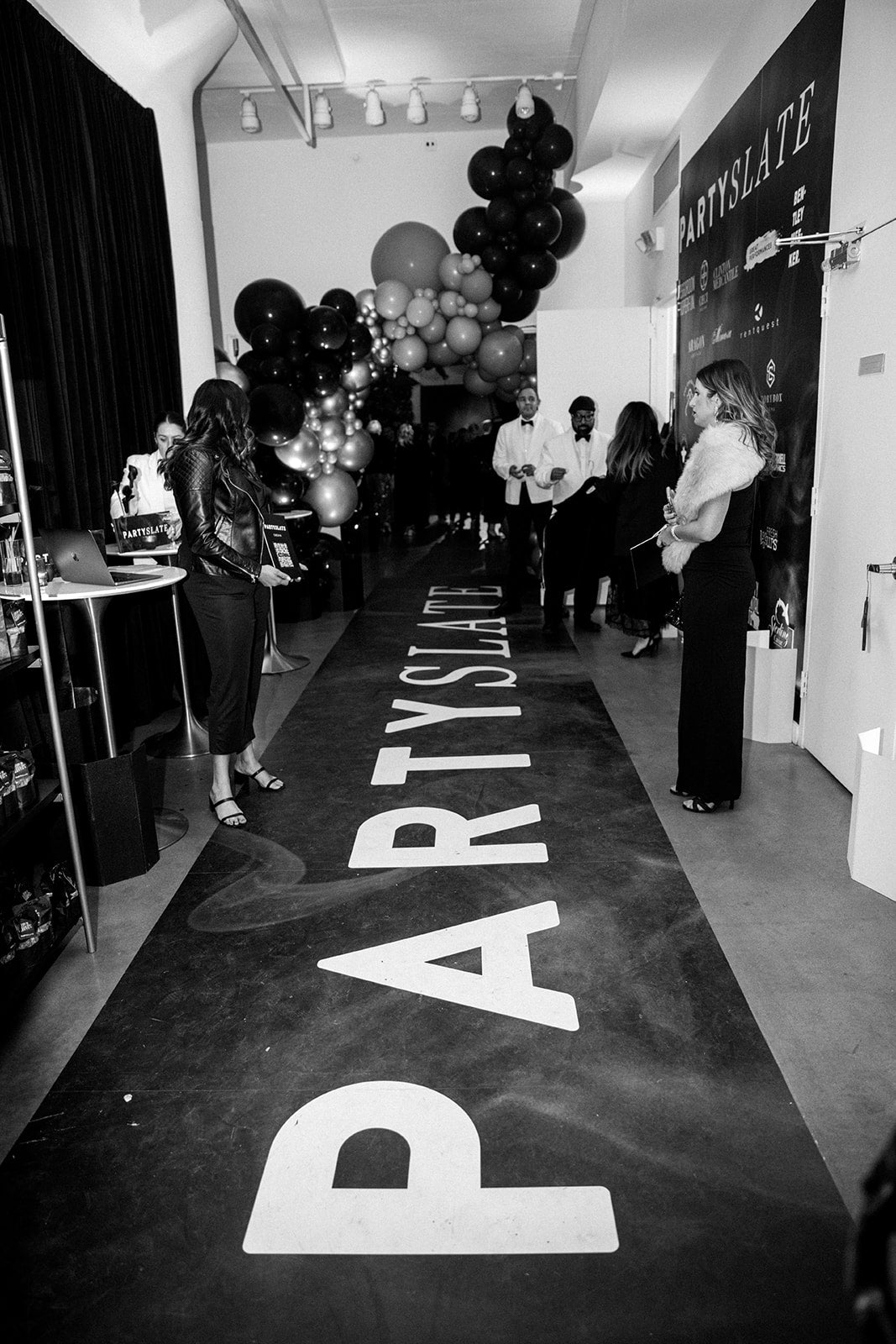This black and white photograph captures the entrance to what appears to be a lively party. The floor features a prominent rug with the text "Party Slate" written in white against a black background. In the foreground, two women stand out in their formal black attire. The woman on the right boasts long hair and dons a luxurious fur wrap around her neck, paired with a long black dress that extends to her toes and high heel shoes. Opposite her, another woman sports a leather jacket, black pants that slightly show her ankles, and stylish dress sandals. The room is bustling with both men and women, adorned with balloons and tables, enhancing the festive atmosphere. A large poster on the right wall also bears the inscription "Party Slate," tying together the theme of the event.